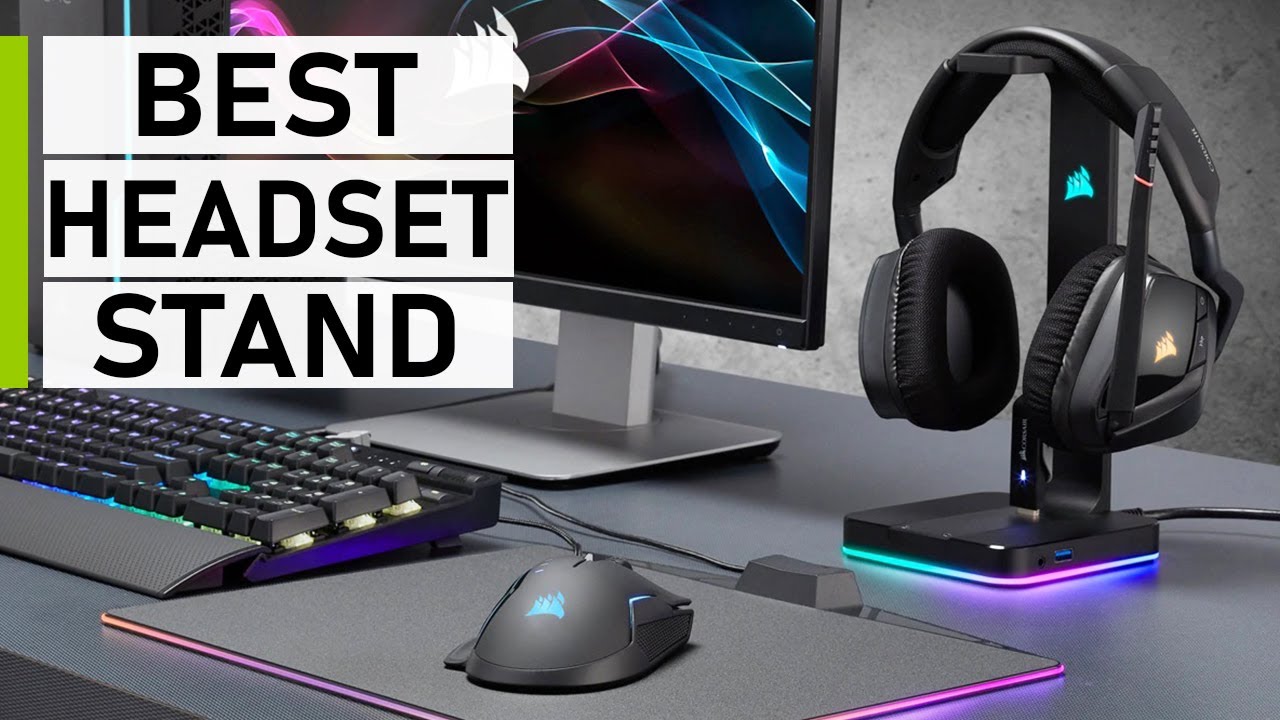The image is showcasing a high-tech advertisement for the "Best Headset Stand." The focal point includes a black headset resting on an elegant stand, both adorned with intricate, abstract images. The stand features subtle blue lights, while the headset's logo shimmers in gold against a backdrop of purple and green lighting. A keyboard and mouse, matching the modern aesthetic with electronic details and cords, accompany the stand. The mouse pad boasts a glowing violet outline, enhancing the visual appeal. The computer screen, partially visible, displays the same abstract image central to the theme, along with bold black letters spelling out "BEST HEADSET STAND" on a clean white background. The harmonious blend of violet, teal, and neon hues ties the ensemble together, creating a sleek and cohesive tech setup.